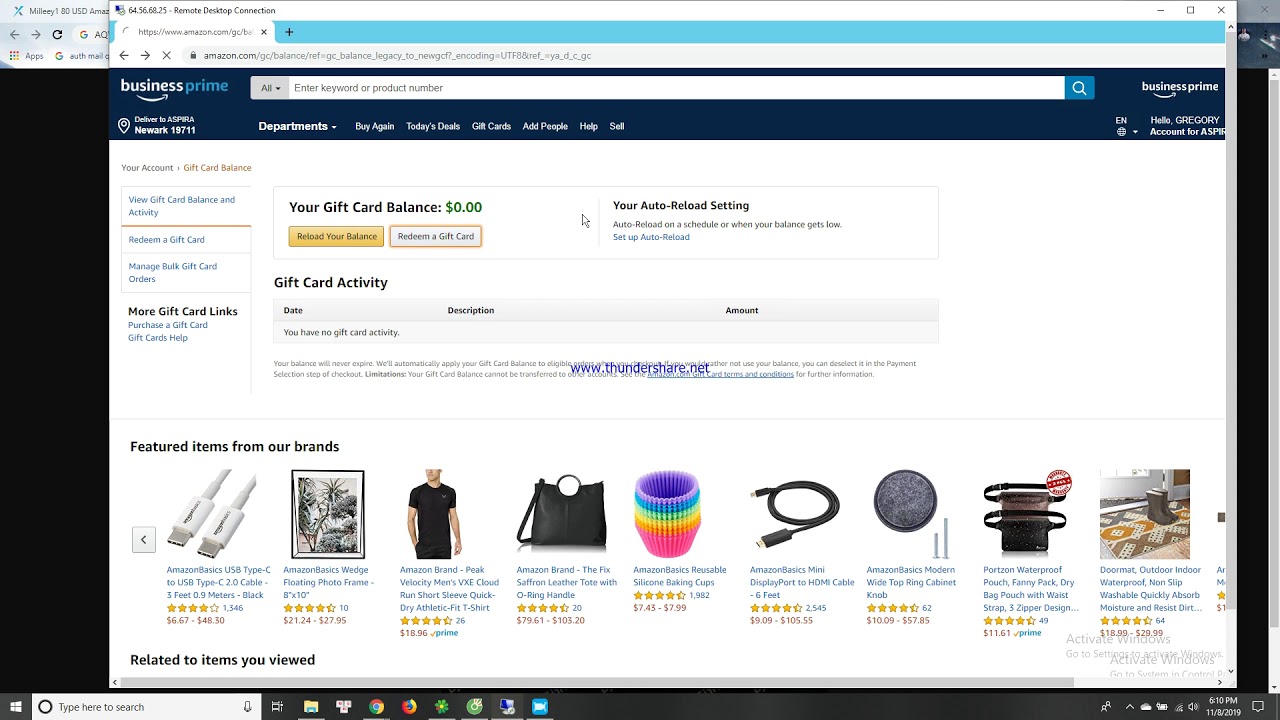Screenshot from Amazon.com gift card balance page. The image displays a current gift card balance of $0.00 in green font. The top menu offers search options for various departments, including featured deals, buy again, gift cards, and an 'All' page. Below the balance, the page showcases "Featured items from our brands" including a phone charger, wall art, a standard black t-shirt, a black tote bag, a stack of silicone cupcake liners, additional phone chargers, some hardware, another bag, and silicone mats. This screenshot captures the interface where users can check their gift card balance, add more funds, or redeem a new gift card on their Amazon account.